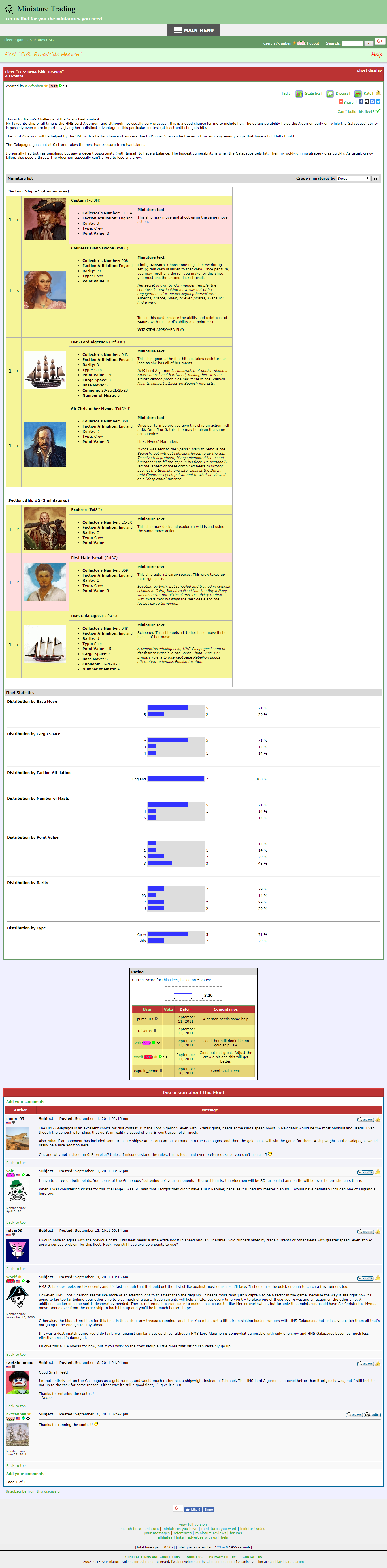A lengthy, heavily distorted screenshot filled with an extensive amount of illegible text and images stretches across the page. Due to the significant resizing, the text has become unreadable, and the images are barely discernable. At the top of the screenshot, a green bar is present. The page is divided into four distinct sections, some of which are headed by red bars. Below one of the red bars, there appear to be instructions. Following this, a segment contains yellow boxes, which likely include questions and answers possibly linked to some obscure images. Among the barely visible images, there is a discernable boat and what appear to be pictures of two men and possibly one woman. Below this section, within the next box, several horizontal blue bar graphs are present, but the text and numbers on them are indiscernible. Further down, a chart can be seen, followed by additional text and images that remain too small to interpret. Despite maximizing the screen, the content remains indistinguishable.